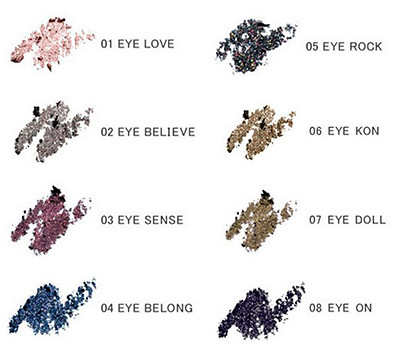The image features eight different shades of eyeshadow arranged in two columns with four shades in each. Each eyeshadow swatch displays a distinct color, marked from 01 to 08, with creative names starting with "EYE" instead of "I." The colors span a diverse palette, including pinks, gold, purple, blue, and black, blending into a visually appealing spectrum. The eyeshadows are named as follows: 

1. "EYE Love" (pink),
2. "EYE Believe" (gray/silver),
3. "EYE Sense" (pinkish-purple),
4. "EYE Belong" (blue),
5. "EYE Rock" (silver),
6. "EYE Con" (gold),
7. "EYE Doll" (brown)
8. "EYE On" (dark purple/black).

The names are displayed next to each color swatch, with the entire arrangement set against a white background, adding a neat, clean aesthetic to the image.